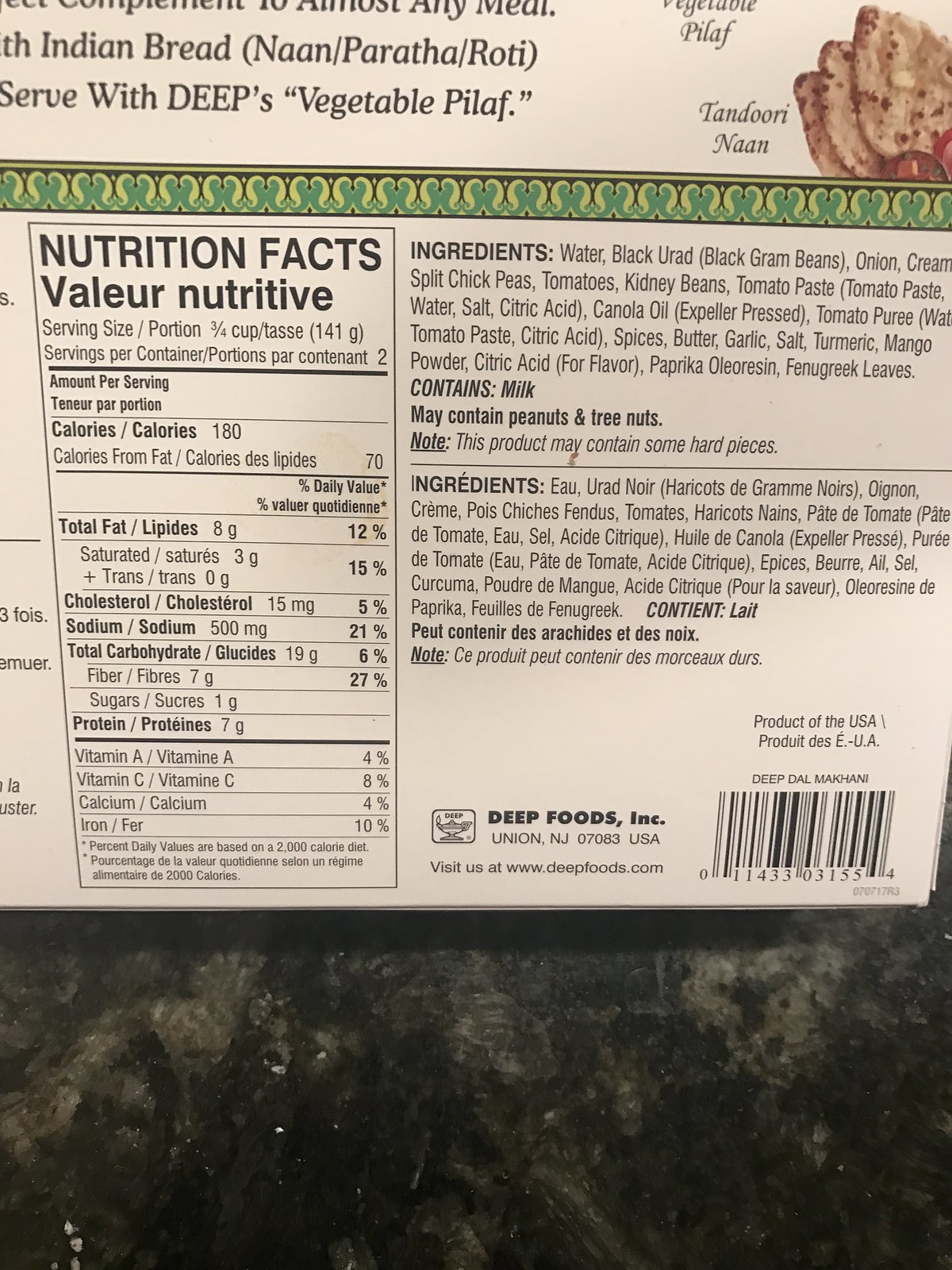The image is a detailed photograph featuring the back of a food product package. The product is identified as a type of Indian bread, although the exact description is partially obscured. Prominently displayed are the nutritional facts, detailing information such as calories, calories per serving, total fat, cholesterol, sodium, total carbohydrates, protein, and various vitamins. Adjacent to these nutritional facts is an ingredients list, which is also provided in French. Additionally, there is a section dedicated to allergens, indicating the presence of milk among other potential allergens. The back of the package also features a barcode and information about the food manufacturer, completing the comprehensive overview of the product details.